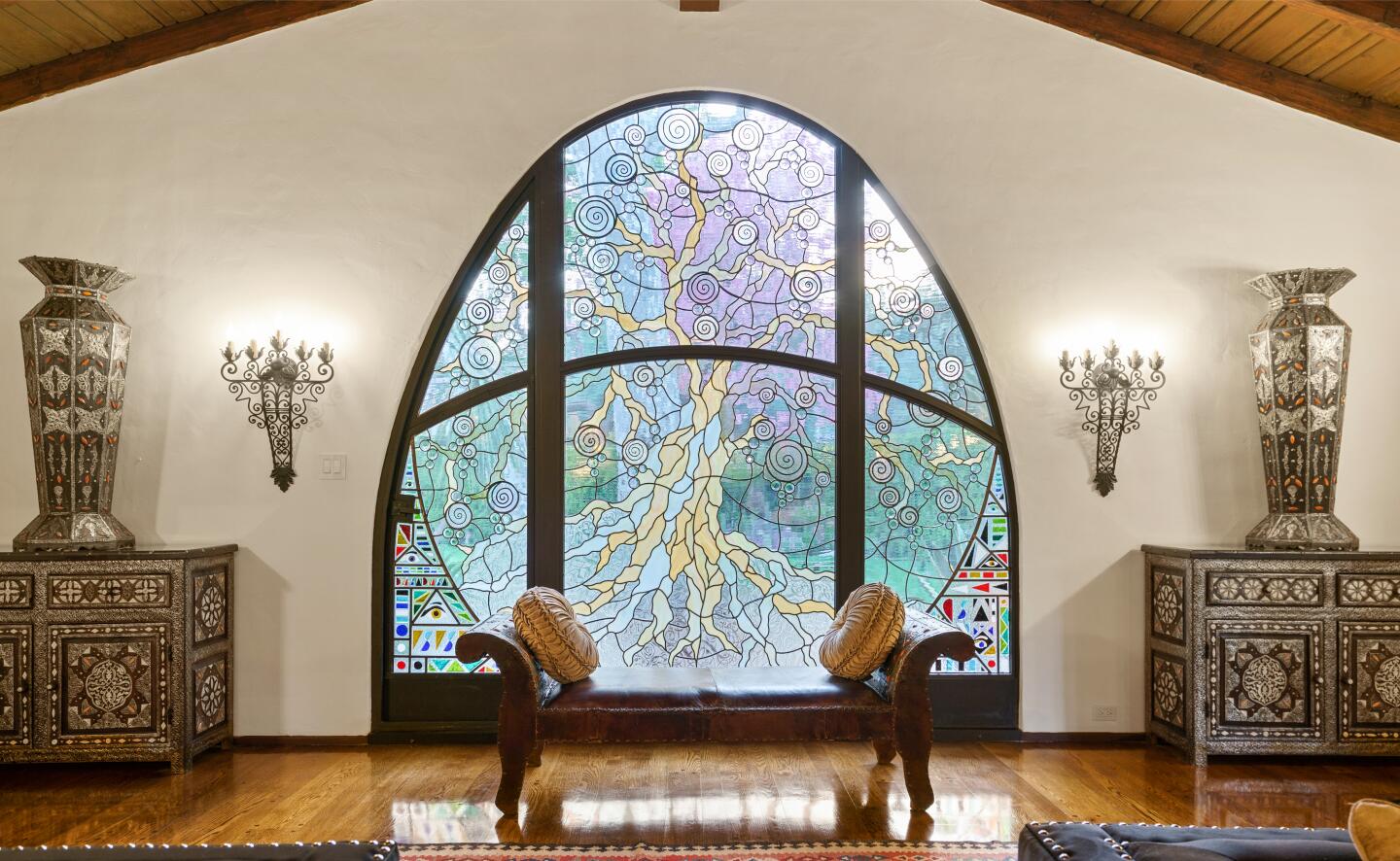The image features a spacious, ornately decorated room characterized by its horizontal-rectangular layout. The focal point of the room is a stunning arched stained-glass window set in the middle of a white-colored wall, detailed with intricate designs that depict whimsical trees adorned with spiral motifs rather than fruit. The stained glass showcases muted hues of lavender, blue, green, yellow, and white, all framed in black.

Flanking the window on either side, the wall is adorned with wrought-iron sconces designed to hold candles. Below these sconces are two highly ornate dressers, each intricately carved and featuring decorative vases on top that mirror the carving details and tan color of the dressers themselves.

In front of the stained-glass window, there is a unique, double-sided bench that mimics the curvature of a Chesterfield sofa’s arms. This bench is upholstered in brown leather and is accessorized with two tan round pillows on each end. The room’s flooring and ceiling are both made of polished, dark wood paneling that adds warmth and cohesion to the decor.